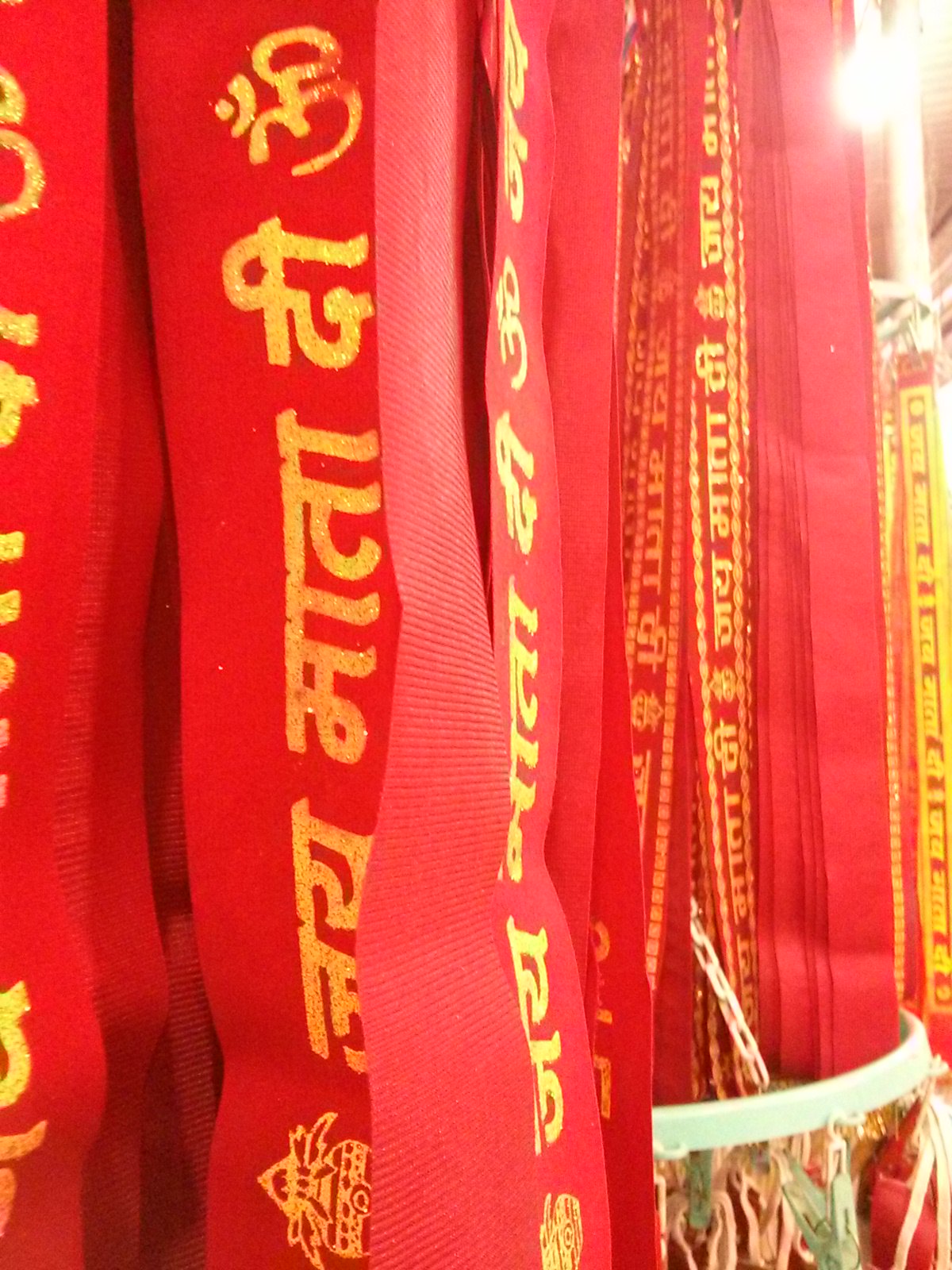This photograph appears to have been taken indoors and showcases an intricate display of numerous red and gold sashes, bands, or banners hanging from the top of the image and extending downwards, with many of them cut off at the bottom edge. Each banner is adorned with gold symbols and writing that resembles Arabic or Asian characters. The scene is densely packed with these vertical streamers, creating a vibrant and elaborate visual effect.

In the bottom right corner, there is a white object that resembles a basket or a circular stand with a chain extending upward into the sashes. This area appears to also have some multicolored elements integrated into the white structure. Additionally, there is a bright light visible in the upper right corner, possibly on the ceiling, and a white stone pillar or pole positioned in front of it. The banners, varying in width from three to five inches, are suspended from the ceiling or another elevated structure, adding to the layered and rich composition of the photograph.